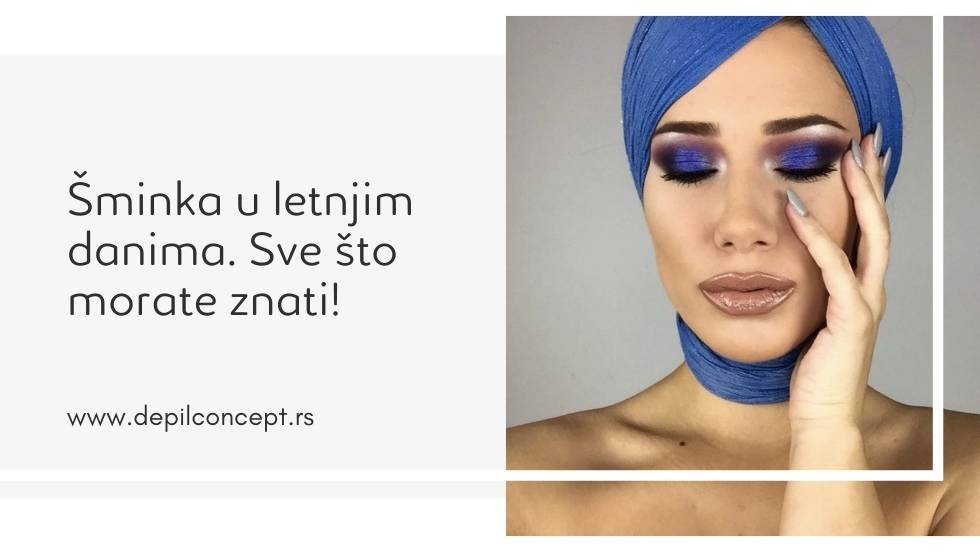The image features a striking portrait of a woman, possibly a model, with her face and shoulders prominently displayed. She is adorned in a dark blue headscarf that wraps elegantly around her neck, partially covering her shoulders. Her eyes are closed, accentuating the vibrant smoky eye makeup with bright blue eyeshadow and dark, thick eyebrows. Her lips are glossy with light brown, shiny lipstick. The woman rests her left hand gently on her left cheek, showcasing long fingernails painted in a light blue or silver-gray color. Her skin tone is a beautiful tan, olive hue. To the left side of the image, there is a grey rectangle with text in a foreign language, and below it, the URL www.depilconcept.rs is visible. The overall scene exudes a sophisticated and serene beauty, with a hint of mystique.